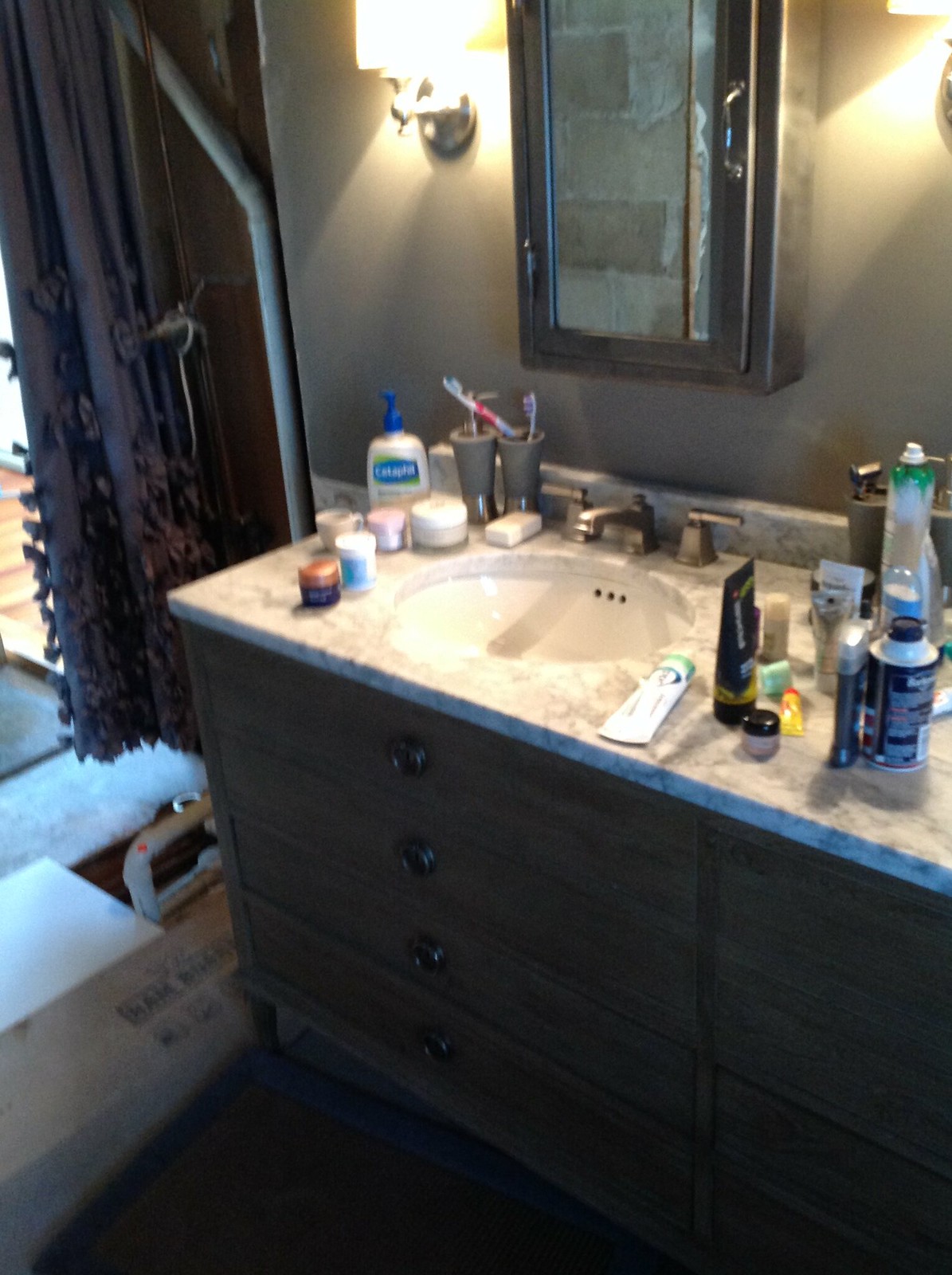This detailed image captures a well-organized bathroom featuring a marble-topped sink with a wooden base. The sink base is adorned with four drawers, each fitted with brass knobs, adding a touch of elegance. The sink itself is a bowl design, equipped with separate hot and cold water knobs. 

On the marble countertop, a variety of items are meticulously arranged. Cylindrical containers filled with makeup products line the area, accompanied by a pump bottle of clear soap. Two conical toothbrush holders sit nearby, each holding a toothbrush—one white with red accents, and the other white with purple accents. 

To the right side of the sink, a collection of skincare products shares space with a stick of deodorant, a can of shaving cream, and a bottle of mouthwash. Additionally, a second deodorant stick is positioned above the sink.

Above the sink, a medicine cabinet fitted with a mirror provides storage and reflection. On either side of the cabinet, two lights illuminate the area, ensuring ample lighting for daily routines. To the left of the sink, the entrance to a walk-in shower can be seen, partially concealed by a hanging shower curtain.